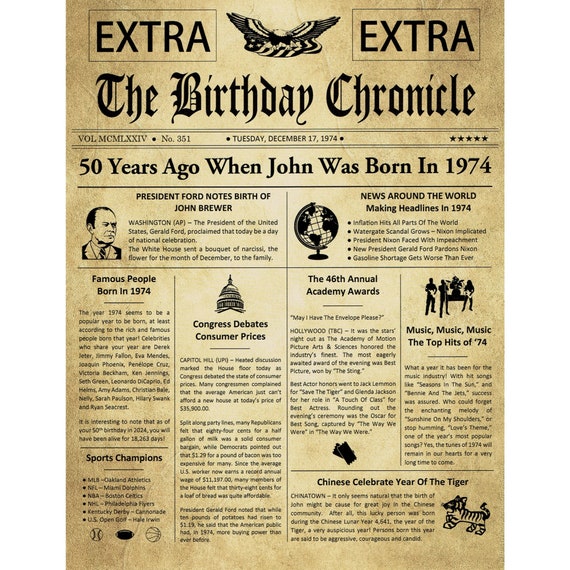The image depicts a novelty newspaper template on a faded yellow background, titled "The Birthday Chronicle," dated Tuesday, December 17, 1974. At the very top corners of the page, the word "EXTRA" is prominently displayed in all caps within black boxes. Below this, in an Old English font, are the words "The Birthday Chronicle." Directly beneath the title, the phrase “50 years ago when John was born in 1974” is highlighted. The layout features two main columns: the left column presents a headline "President Ford notes birth of John Brewer," while the right column details "News around the world making headlines in 1974.” Additional subtitles scattered across the page include "Congress debates consumer prices," "The 46th Annual Academy Awards," "Famous people born in 1974," "Sports champions," and "Music, Music, Music: The top hits of '74," encapsulating the prominent events and details of the year. This design appears to serve as a fun, novelty keepsake likely intended for a birthday celebration.